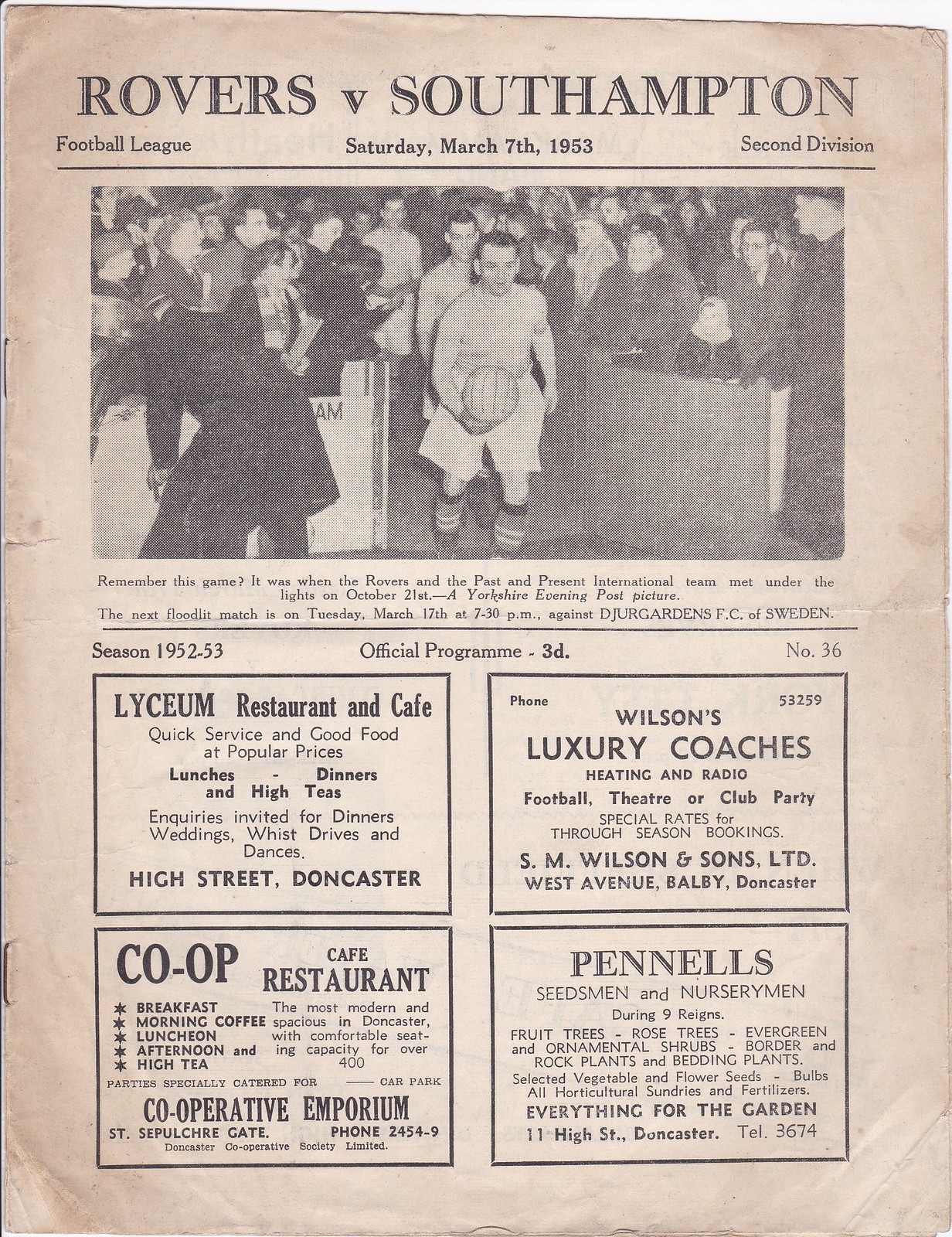The image shows the cover of an old British football programme from the 1952-53 season. The top of the cover features the headline, "Rovers v. Southampton" for a match on Saturday, March 7th, 1953, in the Football League Second Division. Below the headline is a landscape-oriented black-and-white photograph depicting a football team walking onto the field, flanked by a cheering crowd. The captain at the front is holding a ball. Underneath the photo are the words: "Remember this game? It was when the Rovers and the past and present international team met under the lights on October 21st, a Yorkshire Evening Post picture. The next floodlit match is on Tuesday, March 17th, 7.30 pm against Djurgårdens FC of Sweden." Further down, it states, "Season 1952-53, Official Programme, 3D, Number 36." At the bottom of the page are four rectangular advertisements: top left is for Lyceum Restaurant and Cafe, promoting quick service and diverse meal options; top right is for Wilson's Luxury Coaches, offering heating and radio for football, theatre, or club parties; bottom left is for Co-op Cafe Restaurant, emphasizing its modern facilities and large seating capacity; and bottom right is for Pennell's Seedsmen and Nurserymen, advertising a variety of horticultural products.